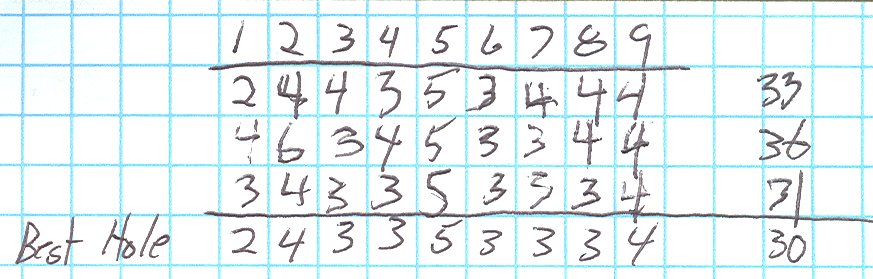The image features a grid of small blue squares on a whitish background, created by intersecting horizontal and vertical blue lines. In the center of this grid, the numbers "1-2-3-4-5-6-7-8-9" are displayed prominently. Below this sequence, four lines of numbers are listed as follows:

- 2-4-4-3-5-3-4-4-4
- 4-6-3-4-5-3-3-4-4
- 3-4-3-3-5-3-3-3-4
- 2-4-3-3-5-3-3-3-4

Each line of numbers is separated by a horizontal line. In the lower left corner of the image, the words "best hole" are written. On the right side of the grid, within some of the blue squares, there are the numbers "33-36-31-30." Notably, there is a line between "31" and "30" that aligns with the lines under the previous sequences of numbers. Additionally, there is a small amount of black coloring at the very top right corner.